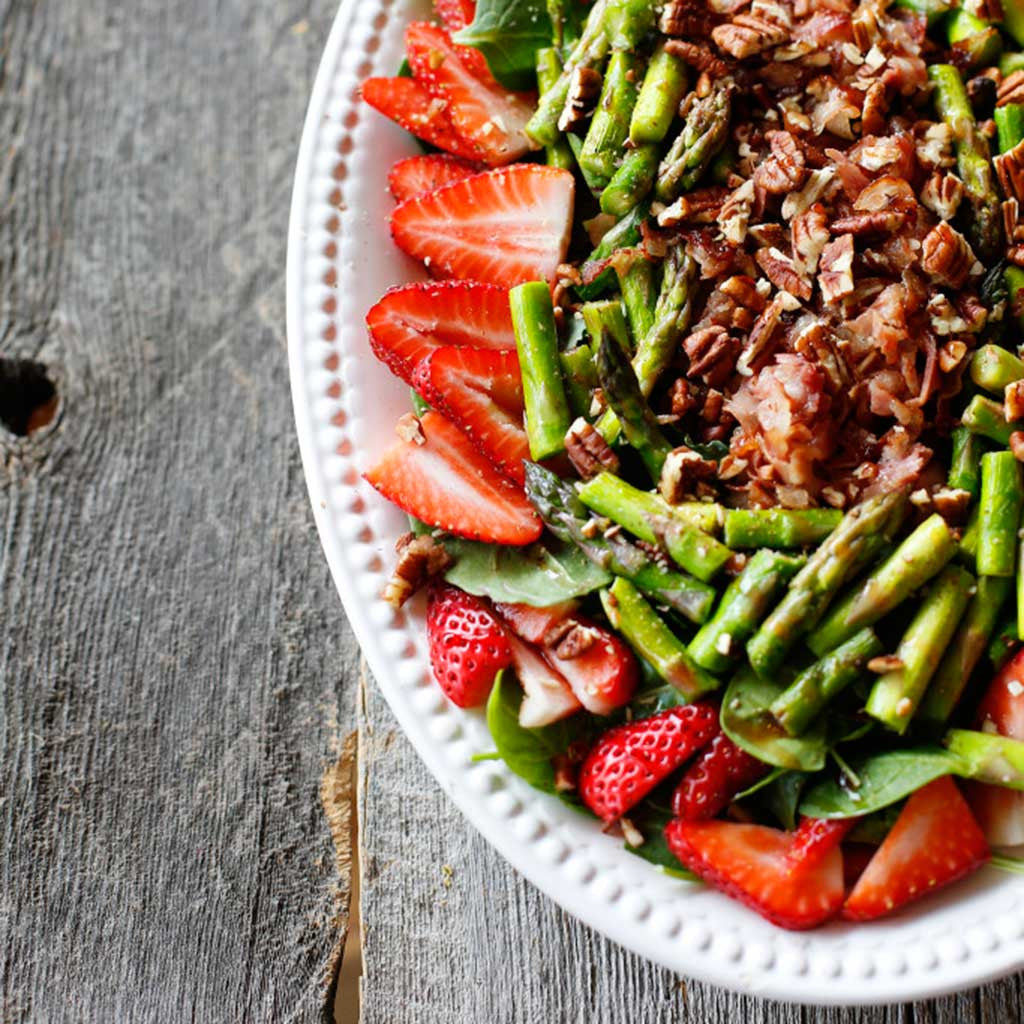This is a detailed close-up photograph of a partially visible white plate with a textured, decorative rim, possibly raised dots encircling the edge. The plate is positioned on the right-hand side of the image, resting on a weathered, grayish wooden plank table that features noticeable imperfections, including a small hole and a crack revealing a tan color underneath.

The plate contains a vibrantly colored, hearty salad composed of fresh ingredients. Around the perimeter of the plate are bright red strawberry halves, showing their seeds and juicy interiors. Mixed within the salad are bright green asparagus pieces, approximately one to two inches long, and crisp green beans. Scattered throughout the dish are crumbled, brown nuts, likely pecans or walnuts, adding a crunchy texture. Additionally, a closer inspection reveals leafy green spinach and potentially some bits of onion. The salad appears to be drizzled with a brown glaze or dressing, which could be balsamic vinegar or olive oil, giving it a glistening finish. The overall presentation suggests a well-made, healthy, and appetizing salad.